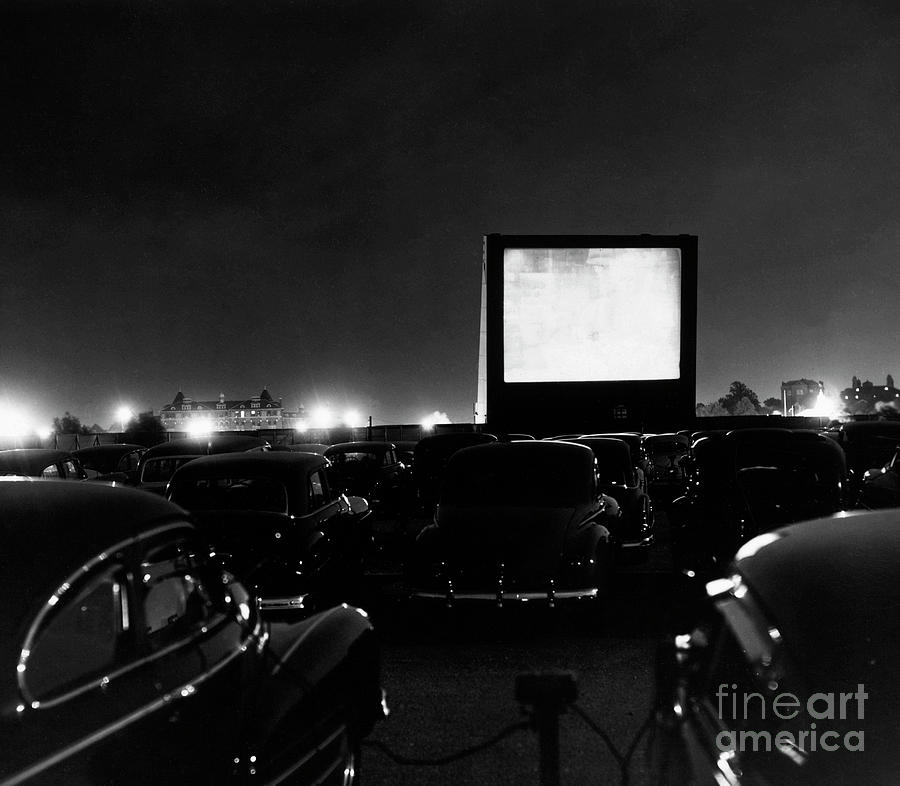This black-and-white photograph captures a drive-in movie theater from the 1950s. The image prominently features rows of classic, rounded hardtop cars with big chrome bumpers, all appearing black due to the monochrome palette. These vehicles are parked closely together in an open lot, facing a large, thick movie screen that stands illuminated but blank. In the foreground, a speaker unit on a pole, with wires running into the car windows, is clearly visible, highlighting the vintage audio setup for listening to the movie. In the distance, the horizon reveals several lighted buildings, including a large house on the left and two more structures on the right. The sky is dark, indicating that the photo was taken at night. The image also bears a watermark from Fine Art America in the bottom right corner.